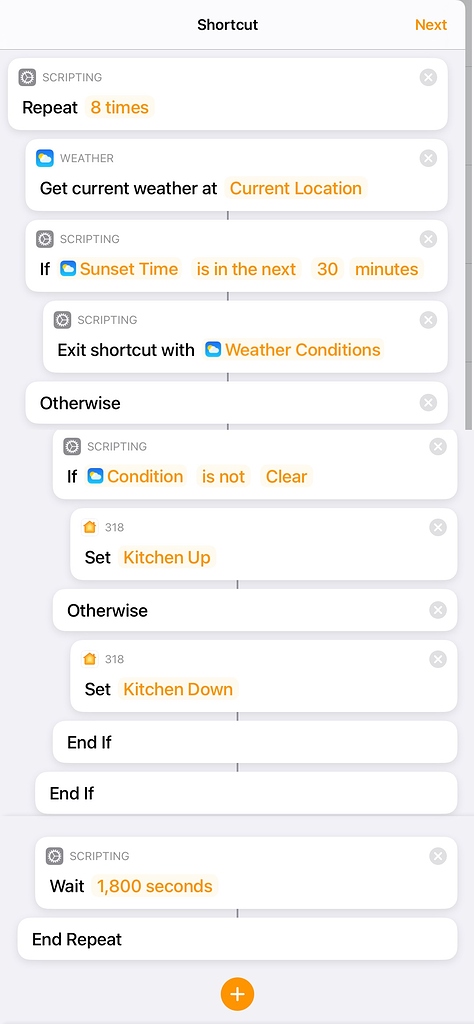A detailed screenshot of a phone display showing an automated scripting workflow titled "Shortcut." The interface presents a series of white boxes laid out against a gray background. The first instruction in the sequence highlights in orange text, "Next, Scripting Repeat 8 times." Following this, a row labeled "Get Current Weather at Current Location" features "Current Location" in orange.

The script continues with an "If" condition: "Weather Sunset Time is in the next 30 minutes," where "Sunset Time is in the next 30 minutes" is highlighted in orange. If this condition is met, the next step is to "Exit Shortcut with Weather Conditions," with "Weather Conditions" also in orange.

For the alternative condition, indicated as "Otherwise," the script checks another "If" condition: "Weather Condition is Not Clear," with "Condition is Not Clear" highlighted in orange. If true, the subsequent action is to "Set Kitchen Up," with "Kitchen Up" in orange. Otherwise, it defaults to "Set Kitchen Down," and "Kitchen Down" is highlighted in orange.

There is a further fallback condition labeled, "And if nothing else." Following this, the script waits "1,800 seconds," with "1,800 seconds" highlighted in orange to signify a 30-minute delay. Finally, the sequence ends with an option to "Repeat." At the very bottom, there is an orange circle containing a plus sign, indicating the option to add more instructions to the script.